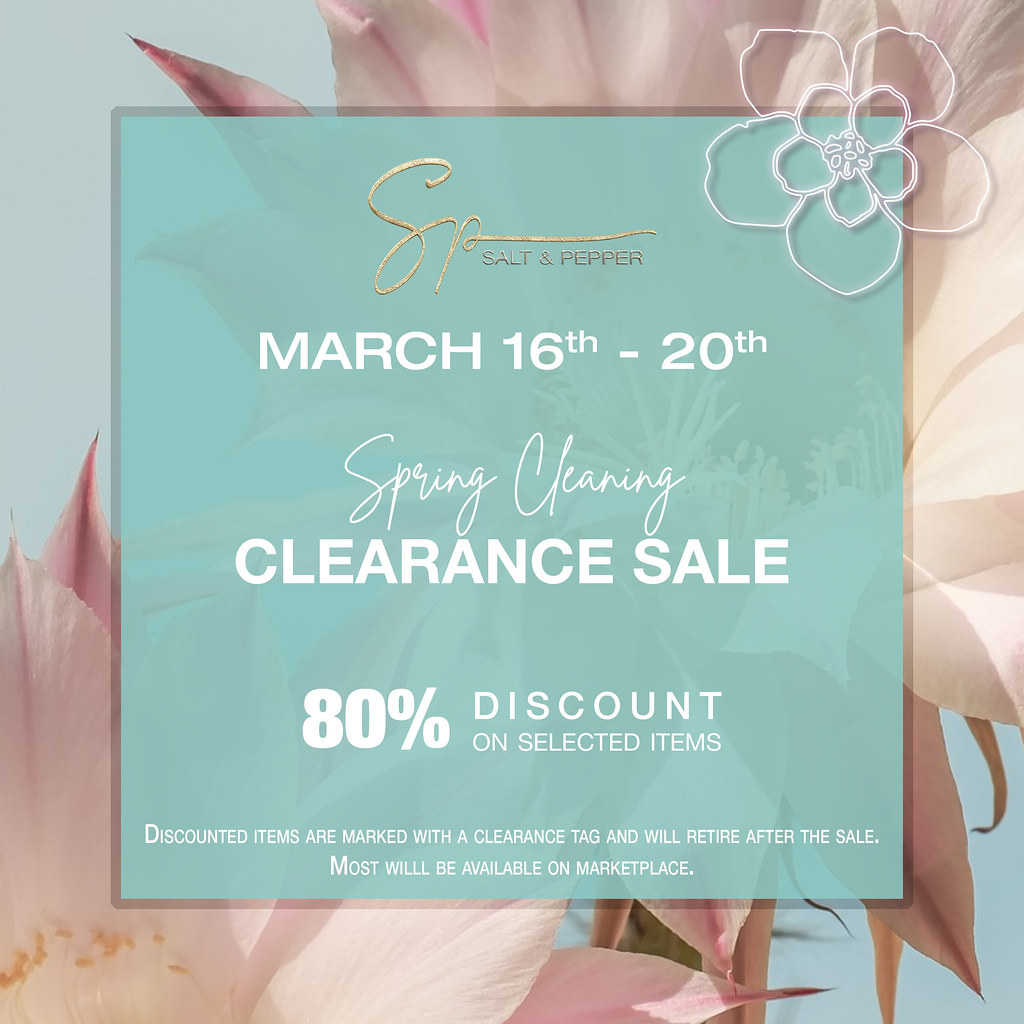The image is a square digital advertisement with a vibrant background featuring a photograph of light pink flowers. One set of petals appears in the bottom left corner, revealing only a part of the flower, while another set showcases the flowers in the top right. Centered over this floral background, there is a transparent turquoise square with a gray border. Within this square, at the top, a golden cursive "SP" logo is displayed, followed by the words "Salt and Pepper" in silver. The text below, written in white font, announces a "Spring Cleaning Clearance Sale" from March 16th to 20th, offering an 80% discount on selected items. Additionally, the right corner at the top of the turquoise square showcases a somewhat neon-looking white flower design. At the bottom of the text, additional details are mentioned: "Discounted items are marked with a clearance tag and will retire after the sale. Most will be available on the marketplace." The cohesive design ties together elements of the pink flower background and a turquoise overlay to create an eye-catching and detailed advertisement.